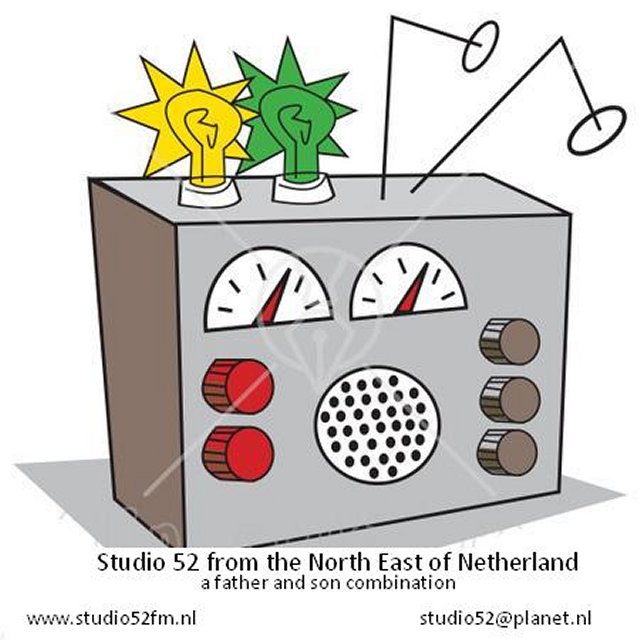The image is a hand-drawn, cartoonish depiction of a large, rectangular gray radio box. On the left side of the radio, there are two red dials, while on the right side, there are three gray dials arranged vertically. In the center of the front face, there is a white circular speaker adorned with black dots. Above the speaker and dials are two gauges with red hands against a white background, positioned such that they resemble eyes. At the top of the radio, there are two antennas flanking two light bulbs—one bright yellow and one bright green. Below this cartoon radio, in black letters, it reads: "Studio 52 from the northeast of Netherlands, a father and son combination." Additionally, there are two websites listed: www.studio52fm.nl and studio52atplanet.nl.